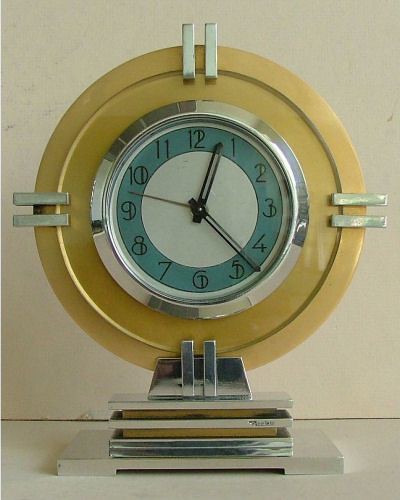The image features an elegant clock resting on a white table against a pristine white wall background. The clock's border is exquisitely crafted from gold, adding a touch of opulence. Notable on the clock face are four pairs of parallel silver rectangles, strategically placed at each quarter section. The clock's base is a sturdy silver structure, supporting the lavish design.

Inside the golden border lies a smaller, refined silver interface housing the main watch face. This watch face is predominantly white, accentuated by an outer blue circle that adds a hint of color. The time is indicated by standard numbering from 1 to 12, meticulously spaced around the face. Two watch hands mark the time: a slender hand points between the 9 and 10, while a slightly thicker hand hovers between the 10 and 12, each contributing to the clock's precise and elegant timekeeping appearance.